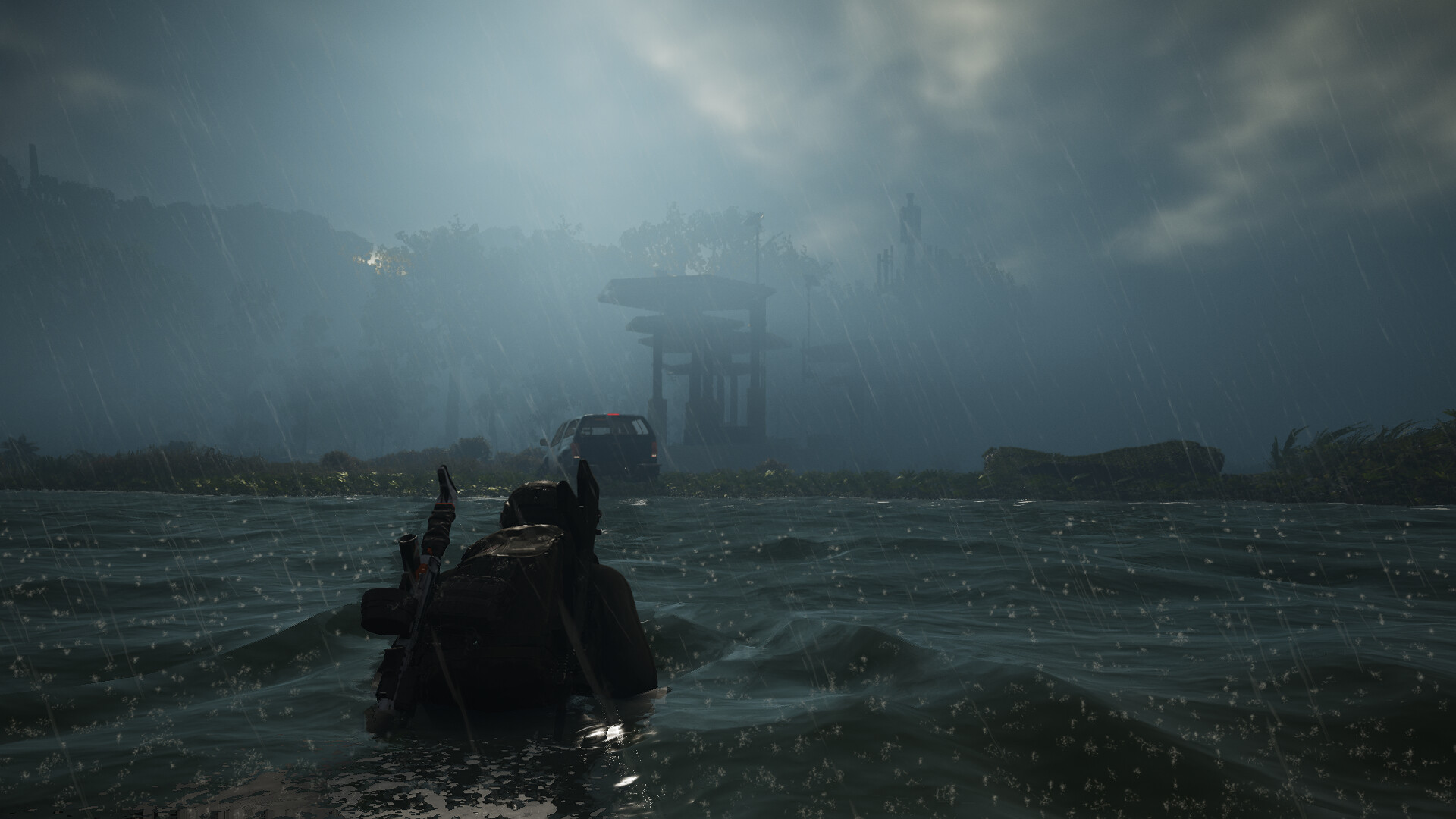A seemingly computer-generated nighttime scene depicts an individual with a backpack trudging through dark, gray-blue water, which is sprinkled with oddly light gray dots, adding to the surreal ambiance. The person's arms are submerged up to the elbows as they navigate towards the background. The landscape transitions at the water's edge, where a vehicle is parked near scattered rocks. Beyond this lies an enigmatic structure comprised of multiple levels and platforms supported by beams. Slightly illuminated in lighter shades of blue and gray, the structure is contrasted by the silhouette of distant trees. To the right, perched on a raised platform, stands the faint silhouette of another figure, adding a sense of mystery and intrigue to the scene.